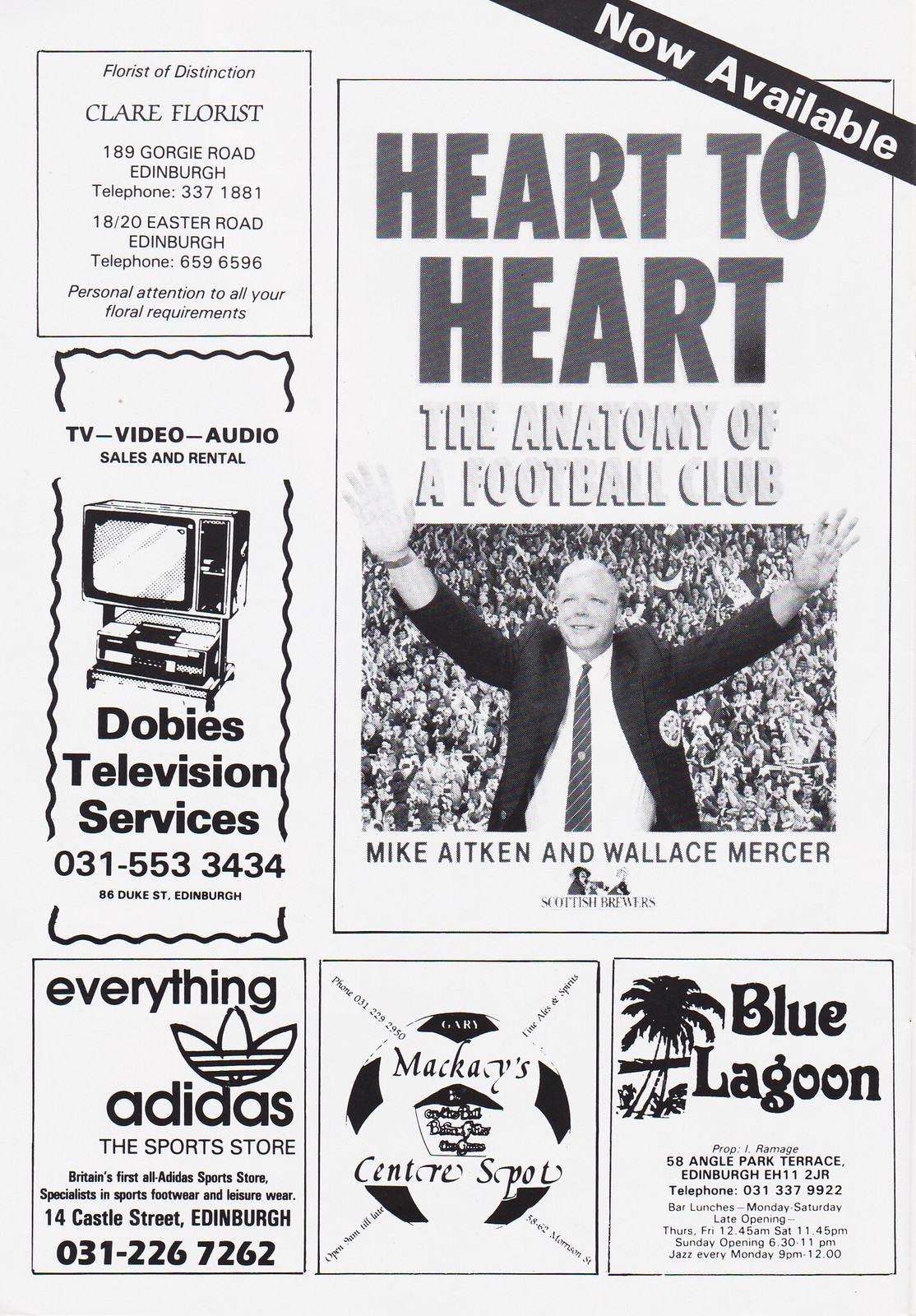This black and white scanned page appears to be from a football program showcasing various advertisements and a feature article. Prominently crossing the top-right corner of the page is a banner reading "Now Available: Heart to Heart, The Anatomy of a Football Club," authored by Mike Atkin and Wallace Mercer, featuring the photo of a balding man in a dark jacket, light shirt, and dark tie, who may be a coach, addressing a crowd. The man's arms are outstretched and he stands before many people, potentially at a football game.

To the left and bottom edges of the page are five distinct advertisement panels. At the top left, an ad for Claire Florist, "A Florist of Distinction," lists two Edinburgh addresses and phone numbers and promises personal attention to floral needs. Below it, Dobie's Television Services advertises TV, audio sales, and rentals, complete with a television graphic and the address 86 Duke Road, Edinburgh. An ad for Adidas highlights Britain's first all-Adidas sports store specializing in sports footwear and leisure wear at 14 Castle Street, Edinburgh.

To the right side of these ads, McKay's Center Spot features a phone number for inquiries. Below McKay's, an advertisement for the Blue Lagoon depicts a palm tree and provides its address at 58 Angle Park Terrace, Edinburgh. It details bar lunch services from Monday to Saturday, along with late and varied opening hours. Additionally, Blue Lagoon offers jazz on Mondays from 9 PM to midnight, suggesting it may be a vibrant nightclub or a restaurant.

Overall, this page merges the elements of a football program with diverse advertisements, reflecting the community and commercial support surrounding the event.